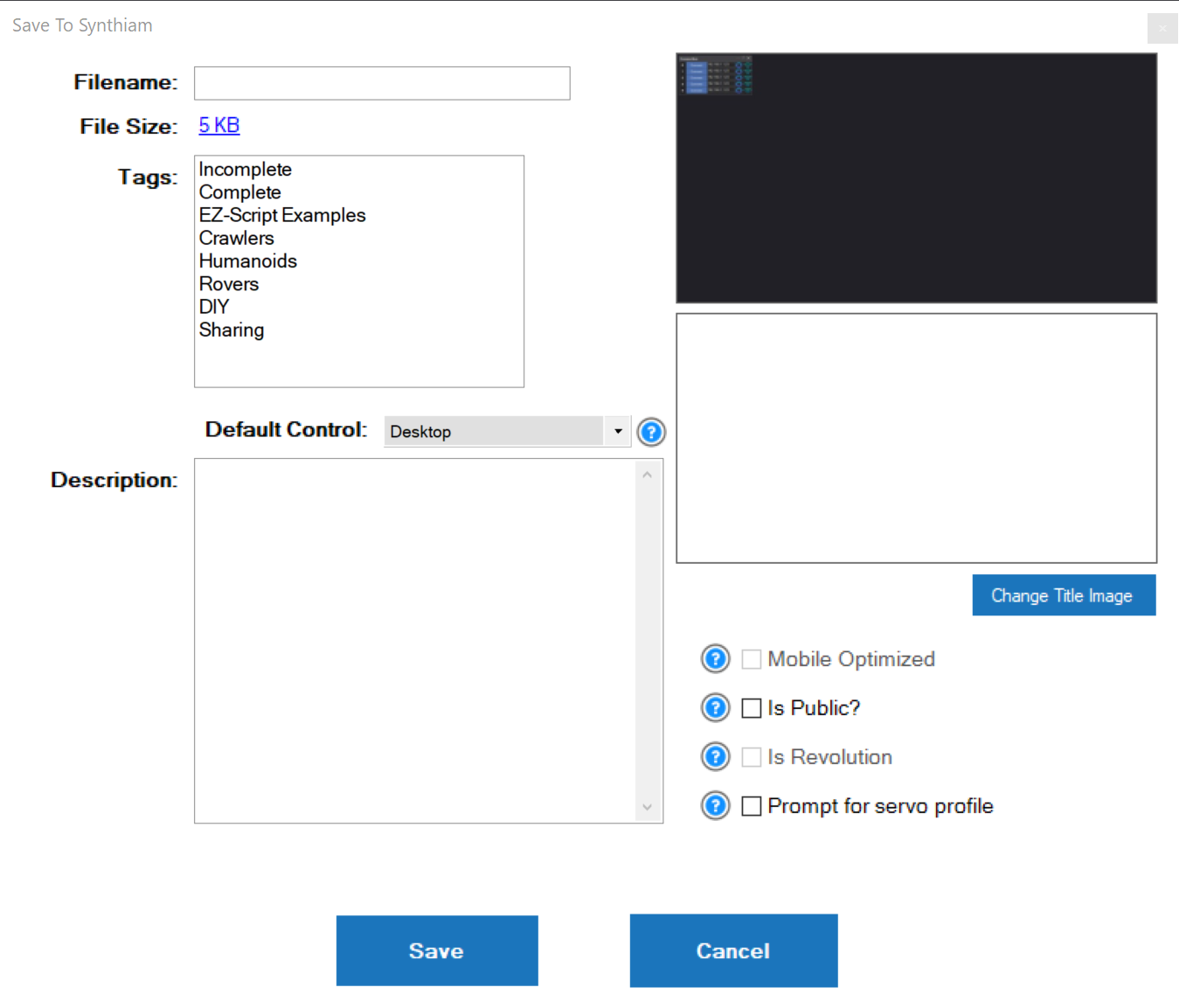**Image Description:**

This appears to be a screenshot of an incomplete file upload or content management system. The interface primarily comprises various options and text fields, detailed as follows:

- **Left Panel:** There’s a section labeled "Save to synthium," though the meaning is unclear. Underneath, there is a label for the file name, which is currently blank. The file size is listed as five kilobytes, which seems unusually small for an image file. Tags associated with the file are visible, including "incomplete," "complete," "easy script examples," "crawlers," "humanoids," "rovers," "DIY," and "sharing."

- **Middle Panel:** The description box is currently empty, and there is a default control desktop label present. Below this, a broken screenshot is mostly black with some blue coloring in the upper left corner, possibly indicating a user interface element for stat tracking. Another blank section is visible underneath.

- **Right Panel:** Several options with checkboxes are visible but none are selected. These options include:
  - "Change tile image" (indicated by a question mark in blue),
  - "Mobile optimized" (unselected),
  - "Public" (unselected),
  - "Revolution" (unselected),
  - "Prompt to server profile" (unselected).

At the bottom of the panel, there is a blue box with white text offering the options to "Save" or "Cancel."

Overall, the system seems designed for uploading and managing files, but the current state suggests that the process is incomplete. The listed file size of five kilobytes is particularly suspicious as it is too small for an image file, indicating a possible error.